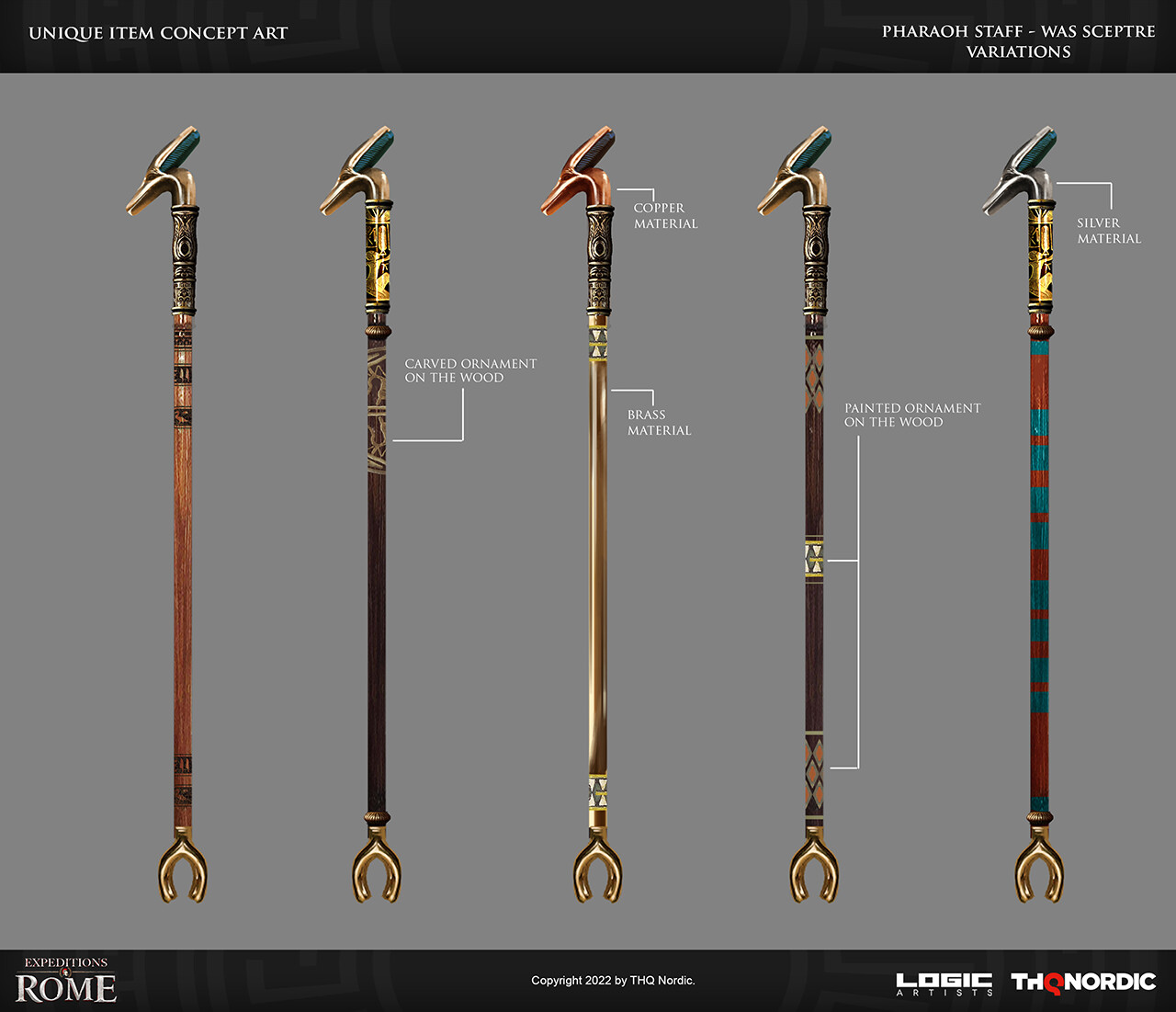The image showcases a collection of five uniquely designed scepters against a grey background. The top of the image features a black banner with the title "Unique Item Concept Art" on the left side and "Pharaoh Staff with Scepter Variations" on the right. Each scepter shares a common structure, characterized by a handle resembling an ibis head at the top and a claw-like fork at the bottom, reminiscent of an upside-down horseshoe, all made of bronze. 

From left to right, the scepters display different colors and patterns: the first is brown, the second is black with brown patterns on the top, the middle one is bronze, the fourth is dark brown adorned with a brown diamond at the top and a green diamond in the middle, and the one on the far right is blue with brown stripes. At the bottom left corner of the image, another black banner reads "Expeditions in Rome," with "Copyright 2022 by THQ Nordic" and "Logic Artist THQ Nordic" in smaller text to its right.